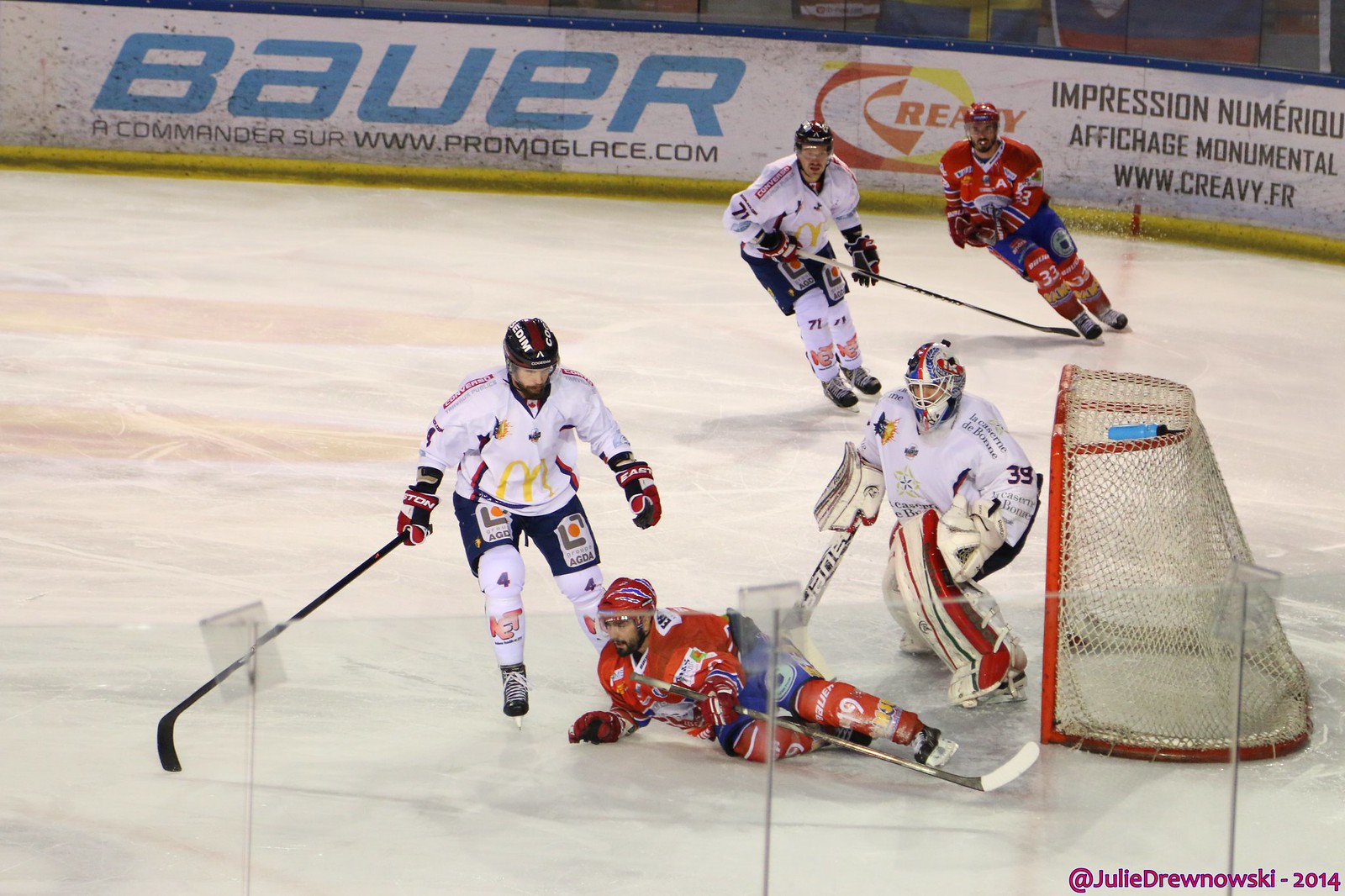In this image, a recreational or lower division hockey game is taking place in an ice rink. The scene features five players, three in white uniforms sponsored by McDonald's—evident from the large "M" on their jerseys—and two in red uniforms. Among the red team players, one is lying sideways on the ice in front of the white team's goalie, who has a water bottle on top of the net. The white team players are donned in white socks, knee pads, blue shorts, and hold hockey sticks like all players. The rink's surface appears worn from use, and a yellow border lines the bottom of the dirty white wall in the background. A prominent white sign on this wall advertises "Bauer" in blue text, positioned above a URL. The goal, trimmed in red and featuring a white net, is situated to the right edge of the image. In the bottom right-hand corner, purple text credits the photo to Julie Drunowski, dated 2014.